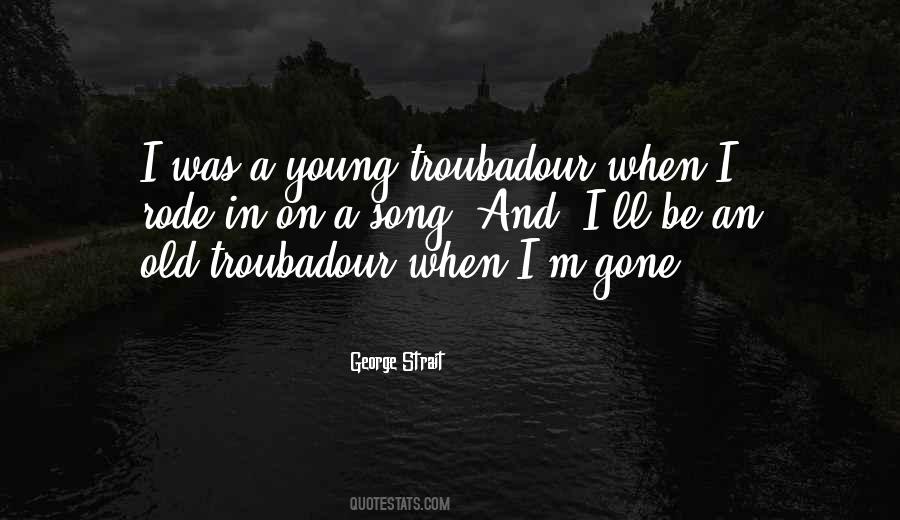The poster features a prominently displayed quote in white script that reads, "I was a young troubadour when I rode in on a song. I'll be an old troubadour when I'm gone," attributed to George Strait and sourced from Quotestats.com. The text is centered on the image, creating a focal point that draws immediate attention. Behind the words, the background is darkened, but if examined closely, reveals a grayscale scene of a river or canal flanked by grass and trees. On the left side, there are a few buildings, potentially including a church or castle with a steeple, enhancing the eeriness of the setting. The cloudy sky above casts a moody atmosphere over the entire scene, adding depth and intrigue. This thoughtful composition appears to be designed for sharing on social media, blending a poignant message with a hauntingly beautiful backdrop.